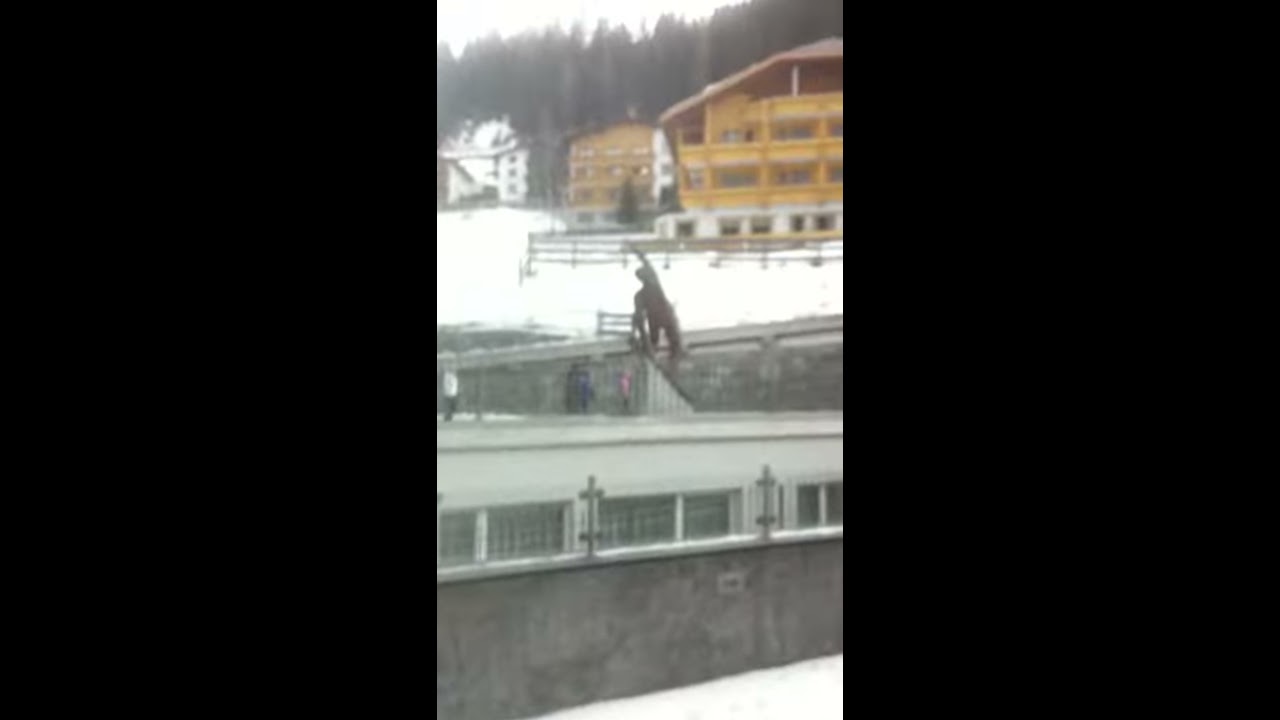The photograph captures a snowy winter scene featuring a pathway bordered by a metallic fence that stretches from left to right across the image. Beyond the snow-covered ground, several large buildings are visible, including a prominent gray and white three-story structure with numerous windows. This building is enclosed by a fence and stands beside a white and brown house. In the distance, another sizable building, possibly a hotel or lodge, can be seen, with a cluster of tall trees providing a natural backdrop. Adding a sense of intrigue, a solitary figure appears to be climbing a stairwell near the foreground, surrounded by the serene, snow-laden environment. The overall ambience is quiet and mysterious, with no other people or vehicles present to disturb the tranquility of the winter landscape.